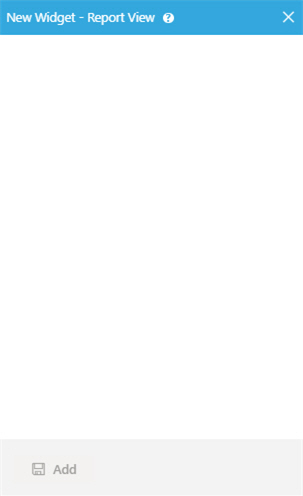This image depicts a screenshot from a cell phone displaying a user interface likely from an app or website page. At the top, a blue horizontal bar spans the width of the screen. Within this bar, the text "New Widget / Report View" is prominently displayed in white. Adjacent to this text, there's a small circular icon containing a white question mark, suggesting help or information is available. On the far right edge of the blue bar, a white 'X' icon is visible, likely serving as a close or exit function.

Below this, the majority of the screen is dominated by a blank, white space, indicating that the main content or webpage is either loading or currently blank. At the bottom of the screen, a light gray rectangular bar extends across the width. On the left side of this bar, there is an icon resembling a square disk, possibly indicating a save function. Next to this icon, the word "Add" is written in bold, gray letters, suggesting an option to add content or items. The interface elements seem to float without distinct borders connecting the top and bottom bars, giving a minimalist and clean design impression.